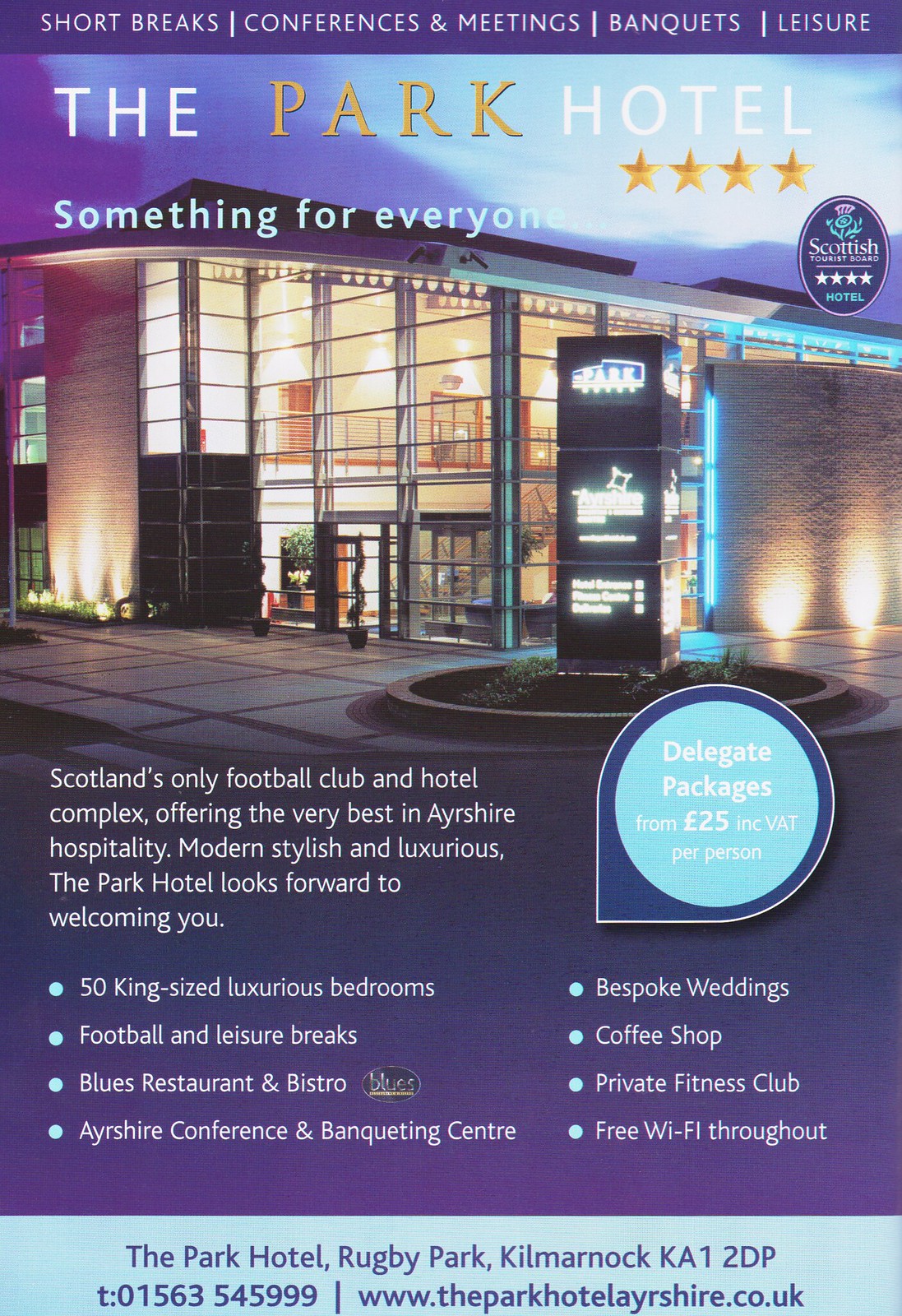The image is an advertisement for The Park Hotel, prominently featuring its name in white and gold letters. The top of the poster includes a purple bar with bold white text delineating various offerings: "Short Breaks," "Conferences and Meetings," "Banquets," and "Leisure." The hotel itself is depicted as a two-to-three story building with large, rectangular windows and a glass front. The facade features the four-star rating prominently beneath the hotel’s name. 

The text emphasizes the hotel's status as "Scotland's only football club and hotel complex offering the very best in Ayrshire hospitality," and highlights its modern, stylish, and luxurious amenities. The Park Hotel boasts 50 king-size luxurious bedrooms, a football and leisure break package, the Blues Restaurant and Bistro, an Ayrshire conference and banqueting center, bespoke wedding services, a coffee shop, a private fitness club, and free Wi-Fi throughout the premises. The advertisement is completed with practical information about the hotel's address, phone number, and website in a light blue bar at the bottom.